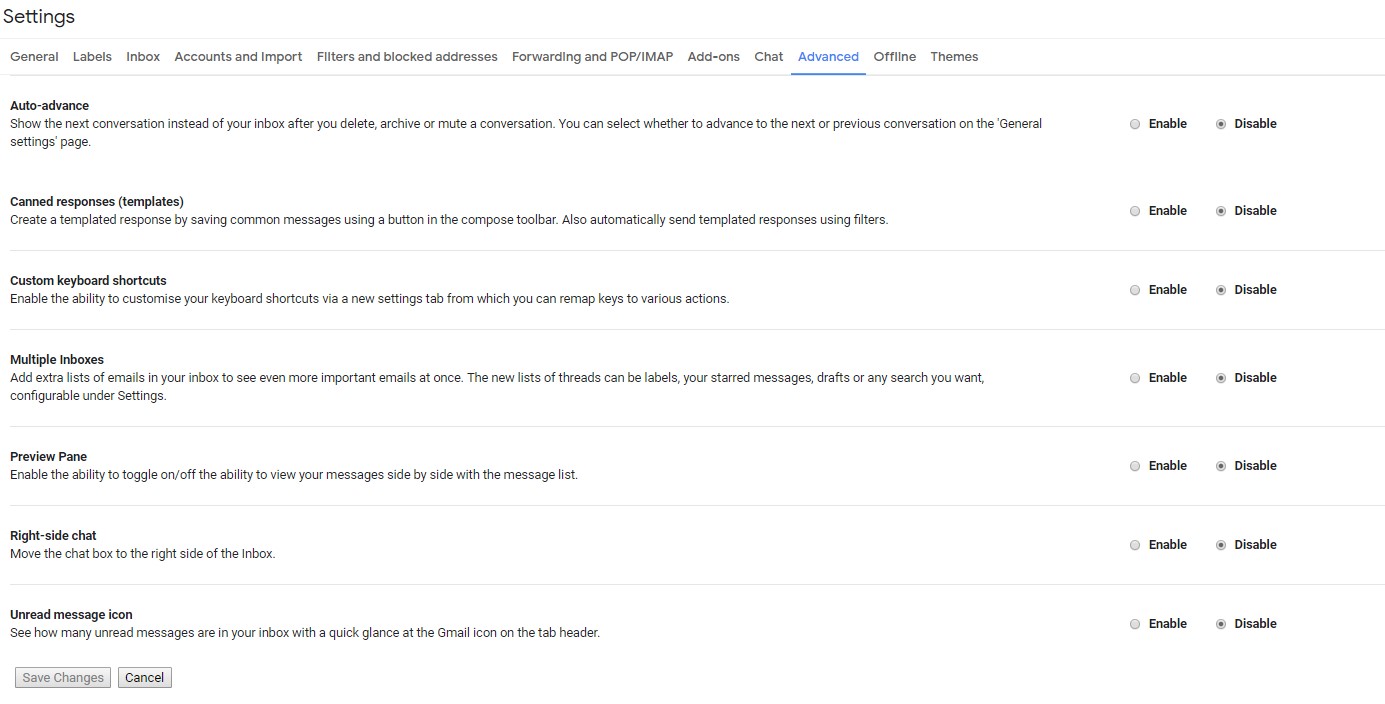The image showcases a user interface with a white background, featuring a navigation menu on the left side. At the top of this menu is the heading "Settings," and beneath it, a list of options: General, Labels, Inbox, Accounts and Import, Filters and Block Addresses, Forwarding and POP/IMAP, Add-ons, Chat, Advanced, Offline, and Themes. 

On the main section of the interface, detailed descriptions for different settings categories are visible. The "Auto-Advance" section allows users to specify whether they want to advance to the next or previous conversation after deleting, archiving, or muting an email. It informs users that this setting can be adjusted on the General Settings page.

The "Canned Responses (Templates)" section explains how to create templated responses by saving common messages using the button in the Compose toolbar. Additionally, it mentions the possibility of automatically sending these templated responses using filters.

Under "Custom Keyboard Shortcuts," it highlights the ability for users to enable and customize keyboard shortcuts through a new settings tab, providing the option to remap keys to various actions.

Finally, the term "Multiple Inboxes" appears towards the bottom, suggesting another feature that can be accessed or configured within these settings.